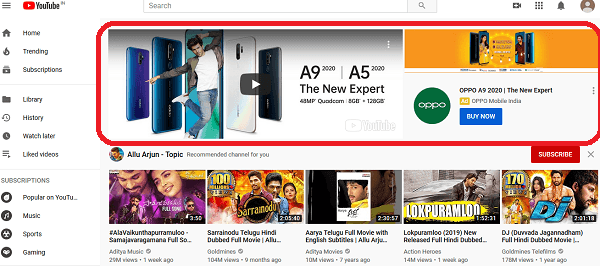This image is a detailed screenshot of an individual's YouTube homepage, prominently highlighting several features. In the top right corner, the recognizable YouTube icon is displayed, while the left-hand side showcases an array of navigational tabs, including Home, Trending, Subscriptions, Library, History, Watch Later, and Liked Videos. Additionally, it lists various categories of the user's subscriptions, such as Popular on YouTube, Music, Sports, and Gaming.

The central section of the screenshot is dominated by a large advertisement for phones, which has been marked with a red outline for emphasis. Below this ad, there is a recommended channel for the user titled "Allu Arjun Topic," displaying thumbnails of five different videos, suggesting diverse content likely related to movies. A red 'Subscribe' button is visible next to the channel name. The recommended videos feature a mix of music and movie-related content, emphasizing the user's interest in cinematic videos.